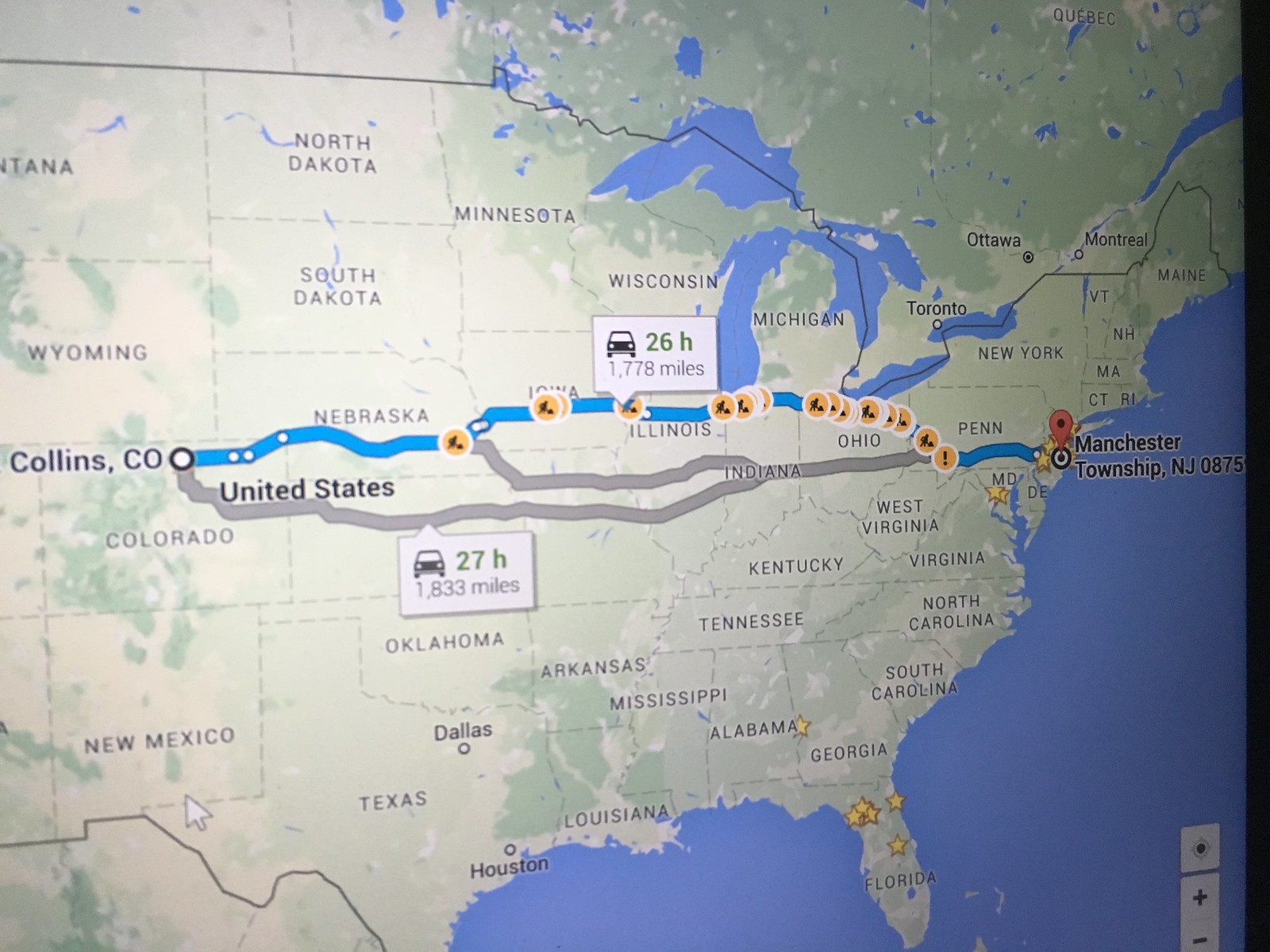This image depicts a detailed map of the United States, extending from parts of Canada on the East Coast, down to the tip of Florida, and over to most of Texas, including half of Montana, Wyoming, Colorado, and New Mexico. The map, which features green landmasses and blue water bodies, labels numerous states including North Dakota, South Dakota, Minnesota, Wisconsin, Iowa, Oklahoma, Arkansas, Mississippi, Louisiana, Alabama, Georgia, South Carolina, North Carolina, Virginia, West Virginia, Kentucky, Michigan, New York, Vermont, Maine, and New Hampshire.

Highlighted on the map is a travel route marked by a bright blue line with yellow circles indicating car positions and speeds. This route depicts a journey starting from Manchester, New Jersey, passing through Pennsylvania, Ohio, Illinois, Nebraska, and ending in Collins, Colorado. There is also a gray line suggesting the return trip. According to the map, the outbound trip covers 1,778 miles in 26 hours, while the return journey covers 1,833 miles in 27 hours. Additionally, the map appears to show Google Maps directions, possibly displayed on a computer or GPS device, with an alternative route slightly to the south marked for comparison. The map features several stars indicating key locations and points of interest along the way.